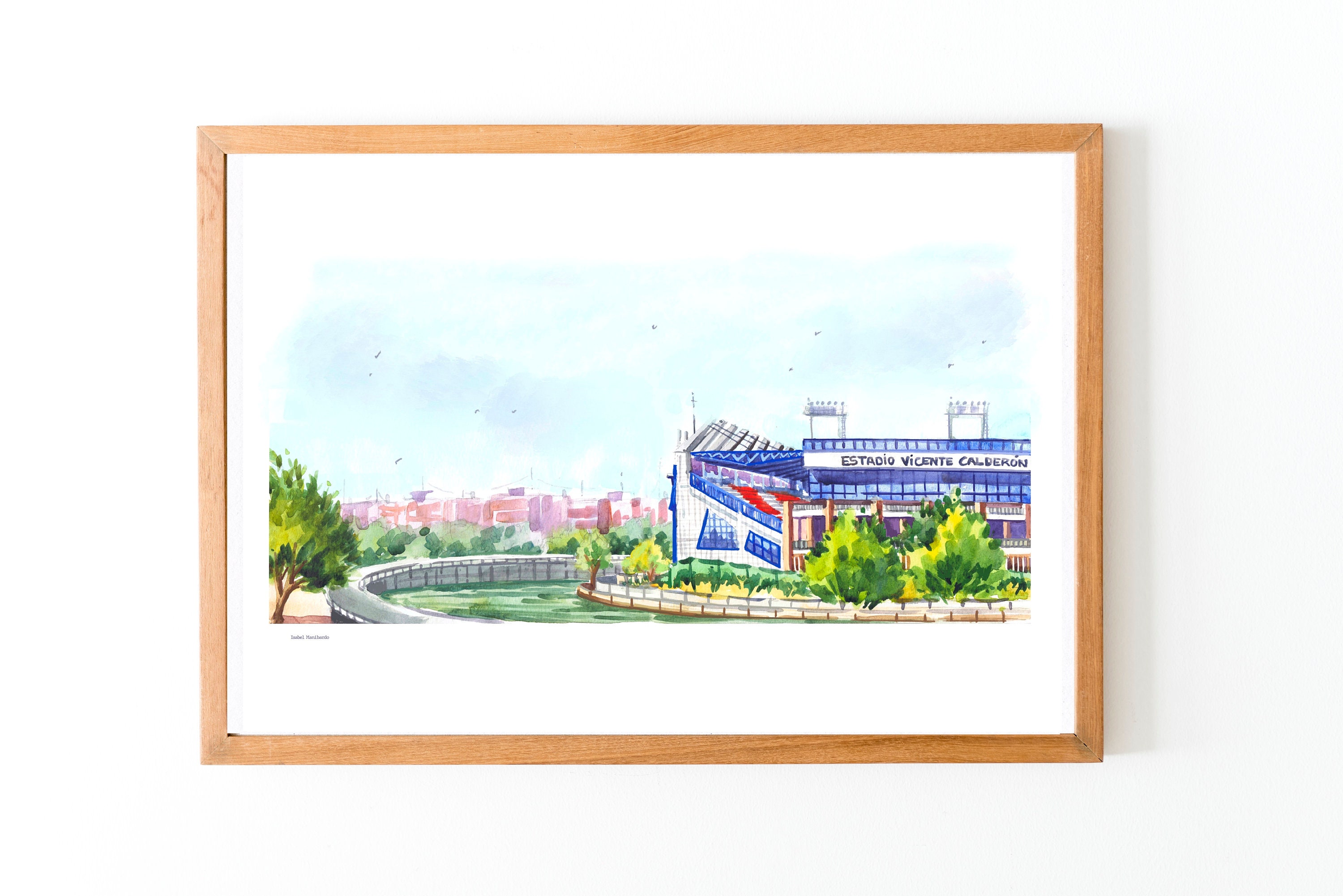This image is a detailed painting, possibly a watercolor or oil-based artwork, framed with a thin, basic wooden frame. The painting itself is centered on a white canvas that extends slightly beyond the edges of the artwork, creating a horizontal rectangle. The scene depicted is an artist's rendition of the Estadio Vicente Calderon, a large soccer stadium. The stadium is prominently blue and white, with red seating and brown pillars, exuding a modern aesthetic. Above the stadium, light towers rise into a blue sky dotted with white clouds. The city in the background includes brown and red buildings that offer a sense of urban context.

In the foreground, the painting shows a lush landscape with several trees, a curved white wall on the bottom left, and a small, white stone or brick wall encircling a group of trees on the right. There is also a waterway with walls surrounding it, adding depth and variety to the scene. Banners hang on the stadium, including a white one extending off the left side of the image. The caption "Estadio Vicente Calderon" is visible on the stadium, and a small print, possibly the artist's signature, is on the left side of the artwork.